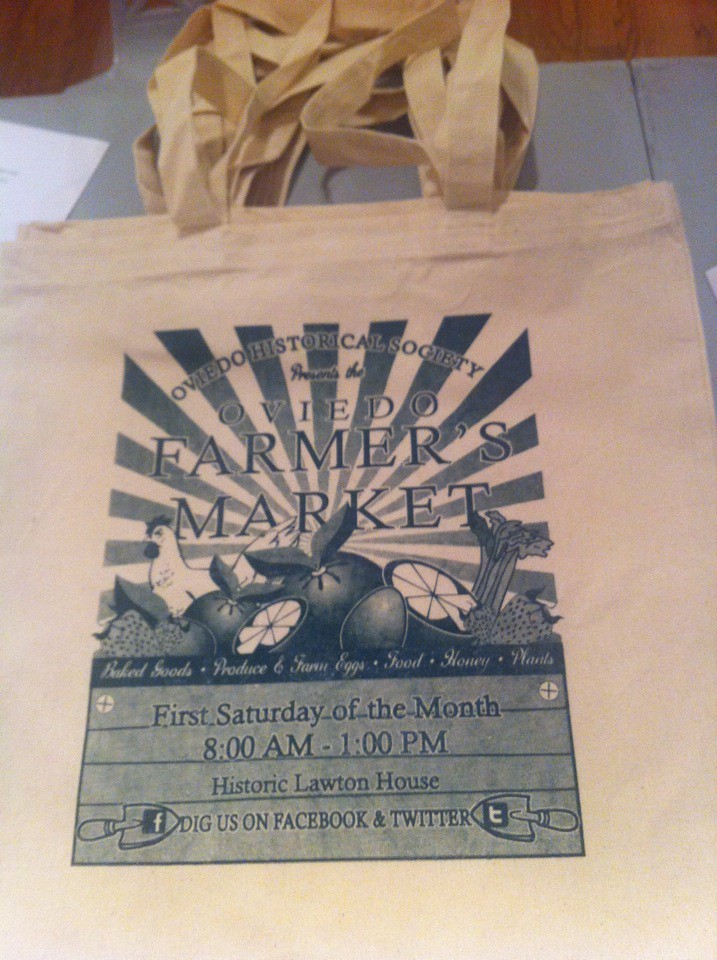This photo features a stack of white cloth tote bags prominently showcasing an advertisement for the Oviedo Farmers Market. Central to the tote's design is a vivid blue and white illustration with radiating sunbeams framing a central image of a white chicken and ripe tomatoes. Above this image, the text reads "Oviedo Historical Cow Society," and just below, it declares "Oviedo Farmers Market." Further down, the text specifies "first Saturday of the month, 8am to 1pm, Historic Lawton House." The bottom of the bag features playful shovels and the phrase "dig us on Facebook and Twitter." Scattered around the bag are illustrations of farm produce and mentions of baked goods, produce, farm eggs, food, honey, and plants. The tote bags lie on a grey wooden floor, in front of a wooden cabinet, with a wooden column to the side and a reddish wooden table in the background. This sturdy tote is perfect for carrying all the fresh goods you can find at the market.